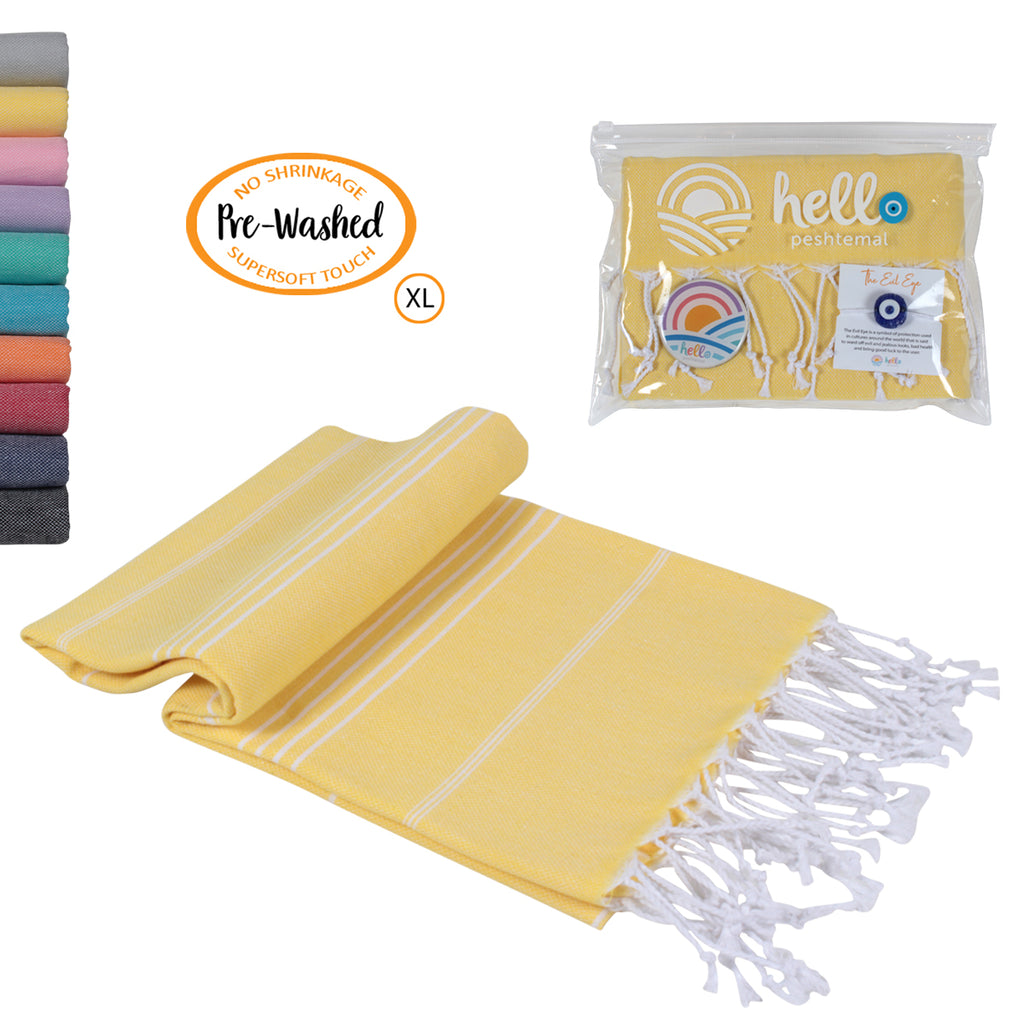The advertisement showcases a folded yellow throw blanket with white horizontal stripes and white fringe, prominently placed against a white backdrop. In the upper left corner, a spectrum of colors available for this blanket, including gray, yellow, pink, purple, green, blue, orange, red, navy, and black, is displayed. Centrally featured is an orange-outlined stamp highlighting key selling points: "No Shrinkage, Pre-Washed, Super Soft Touch, XL." In the top right corner, the product is shown within its clear plastic packaging, labeled "Hello Pestimal."